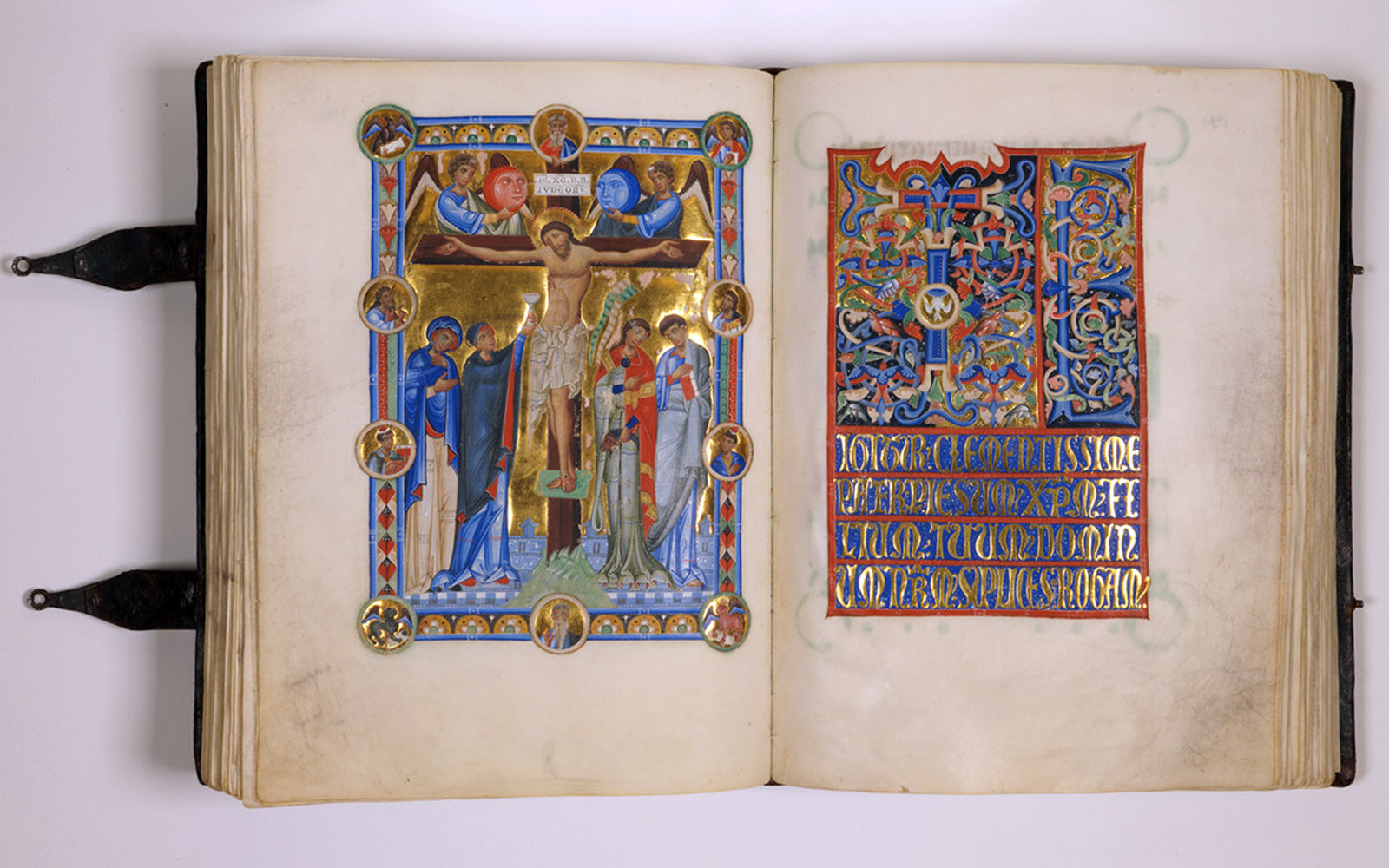The image showcases an old, ornate Bible opened to two vivid pages. The Bible, likely leather-bound, has two visible straps on the left side meant to secure the book closed when not in use. The book rests on a white table, and the photograph captures a top-down view.

On the left page, a richly detailed illustration portrays Jesus on the cross, surrounded by angels at the top and mourners at the bottom. This scene is set against a rectangular blue background, with extensive use of gold, which appears to give the image a glowing effect. Bordering this main image are smaller circular images and intricate designs, adding to the overall ornate appearance.

The right page features a Gothic-style cross embellished with colorful red, blue, and green swirls. Below this, gold-colored text, possibly in Greek, is aligned into four lines, framed by a reddish-orange border and intricate designs above. The gold text and accents on both pages shine, emphasizing the detailed and historical craftsmanship of the book.